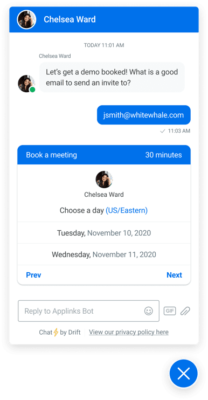A screenshot taken on a mobile device or tablet shows a messaging interface primarily in white and blue tones, with black text. At the top, a blue banner displays a slightly blurry profile picture of a brunette woman, seemingly smiling, next to white text that reads "Chelsea Ward." Below the banner, the current time is specified as "Today at 11:01 a.m." and a green status icon indicates that Chelsea Ward is online. 

A message from Chelsea reads, "Let's get a demo booked. What is a good email to send the invite to?" 

The response, highlighted in blue, states "jsmith@whitewhale.com" and was sent at 11:03 a.m. Following this, a blue banner labeled "Book a Meeting" leads to options for scheduling a 30-minute meeting. Chelsea Ward provides two hyperlinked date options: Tuesday, November 10th, 2020, and Wednesday, November 11th, 2020. Navigation buttons for "Previous" and "Next" are visible at the bottom of the interface.